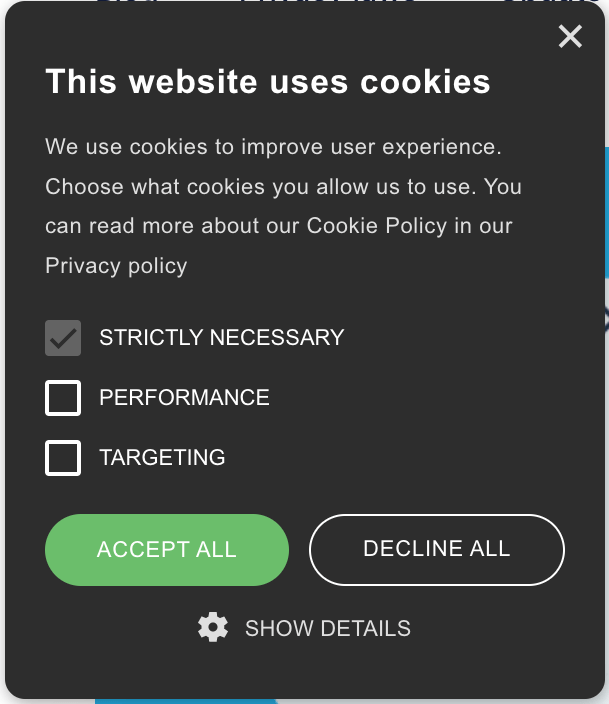In the top right corner of the image lies a prominent gray "X" inside a black box. Just below this, large white lettering reads "This website uses cookies." Directly under this text, in smaller gray font, it states, "We use cookies to improve user experience. Choose what cookies you allow us to use. You can read more about our cookie policy and our privacy policy."

The left side of the image features three distinct lines, each corresponding to different categories of cookies that can be selected. Adjacent to these lines, there is a layout consisting of gray and black squares featuring check marks or borders, alongside descriptive text.

The first line starts with a gray square containing a black check mark. To its right, in capital white letters, the words "Strictly Necessary" are displayed. 

Below this, there's a black square framed with a white border, and to its right, white capital letters spell out "Performance." 

Further down, another similar black square with a white border appears, and next to it, white capital letters read "Targeting."

Towards the bottom of the image, there are two prominent oblong buttons. The first button is green with the white capital letters "ACCEPT ALL." To its right, a black oblong button outlined in white displays "DECLINE ALL" in capital white letters. 

Beneath these buttons, a gear icon is present, with the text "Show details" positioned to its right.